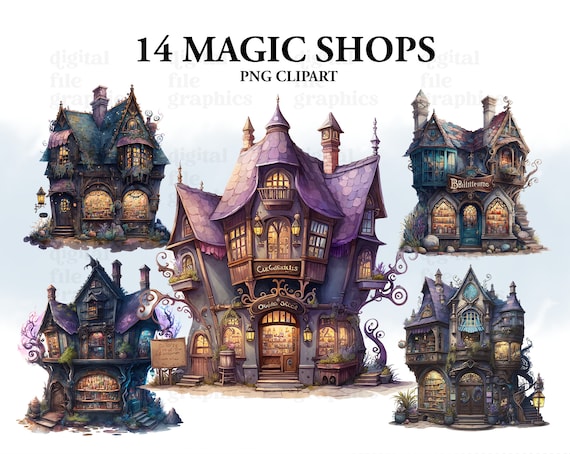The image features a collection of fantasy-themed magic shops, clearly labeled at the top with bold black text reading "14 Magic Shops" and "PNG Clip Art" beneath it. The scene is set against a white background, with a distinct light gray watermark saying "digital file graphic" scattered throughout.

At the center of the image, a prominent multi-storied shop stands out, distinguished by its unique purple roof and lighter-colored walls. This central building exudes an old-school, medieval vibe, complete with wooden windows framed by wooden arch supports. Additionally, it boasts two visible shop signs and appears to have items displayed on shelves inside.

Surrounding the central shop are four other shops, placed in each corner of the image (top left, bottom left, top right, and bottom right). These buildings share a similar fantasy design, characterized by dark, bluish color schemes, tall and sharply angled roofs that give off a slightly haunted feeling. While all are multi-storied, the central and top right shops feature the most visible signage, contrasting with the more discreet signage on the others. Notably, the shop in the bottom left corner has a larger sign positioned to the side rather than above the doorway.